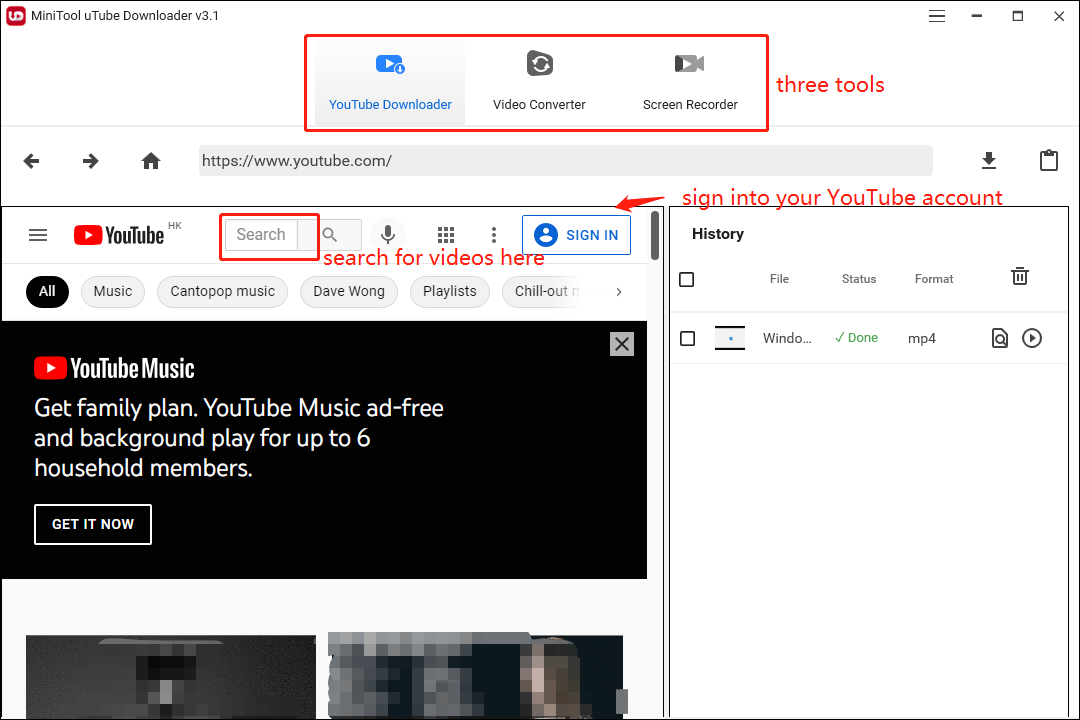The screenshot showcases a webpage with a white background, featuring the interface of "MiniTool YouTube Downloader v3.1." At the top of the page, there's a square emblem with the software name positioned outside the emblem: "MiniTool" (with a capital "M" and "T") and "YouTube" (with a capital "Y" and "TUBE").

To the right, there are three icons: the first with three horizontal lines (middle line darker), a minus sign (to minimize the page), a square (to expand the webpage), and an "X" (to close the page).

In the center, prominently displayed, is the title "YouTube Downloader" in blue, followed by "Video Converter and Screen Recorder," bordered by a red outline. Below this, the text "Three Tools" (spelled out) is visible.

Further down the page, there are navigation arrows (left and right), a home icon, and a web address bar showing "YouTube.com." The main content area displays a portion of the YouTube page with the "YouTube search" bar enclosed in a red square, a search prompt, and a sign-in section highlighted with a red arrow, indicating "Sign into your YouTube account." It also mentions offers such as "YouTube Music Family Plan" and "YouTube Music Ad Free and Background Play for up to six household members."